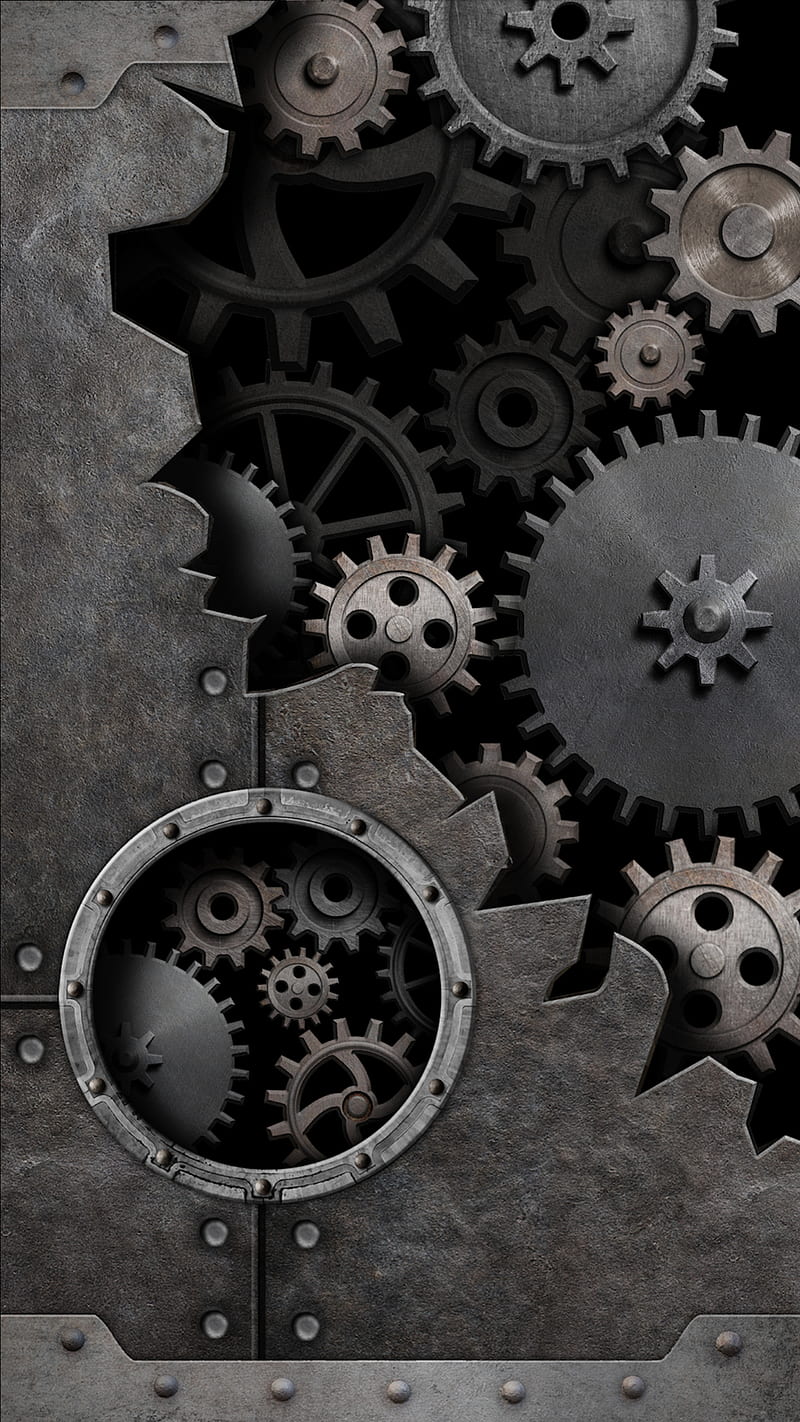This detailed drawing presents an industrial metal scene filled with a variety of intricate gears and cogs. Dominating the image is a rectangular metal area at the bottom, adorned with numerous silver circular bolts. Moving upward, the metal surface continues with bolted sections, featuring jagged, knife-like edges that evoke a sense of sharpness and danger. The top right corner reveals a torn steel plate with exposed inner workings, showcasing an array of interconnected gears of varying sizes. These gears range from tiny to large, with designs that include circular centers and multiple holes, all rendered in shades of silver and gray. A noticeable feature in the lower left-hand corner is a porthole window encircled by a shiny metal ring and rivets, offering a glimpse of additional gears inside. These internal gears possess similar shapes and styles, further emphasizing the intricate complexity and industrial nature of the scene.